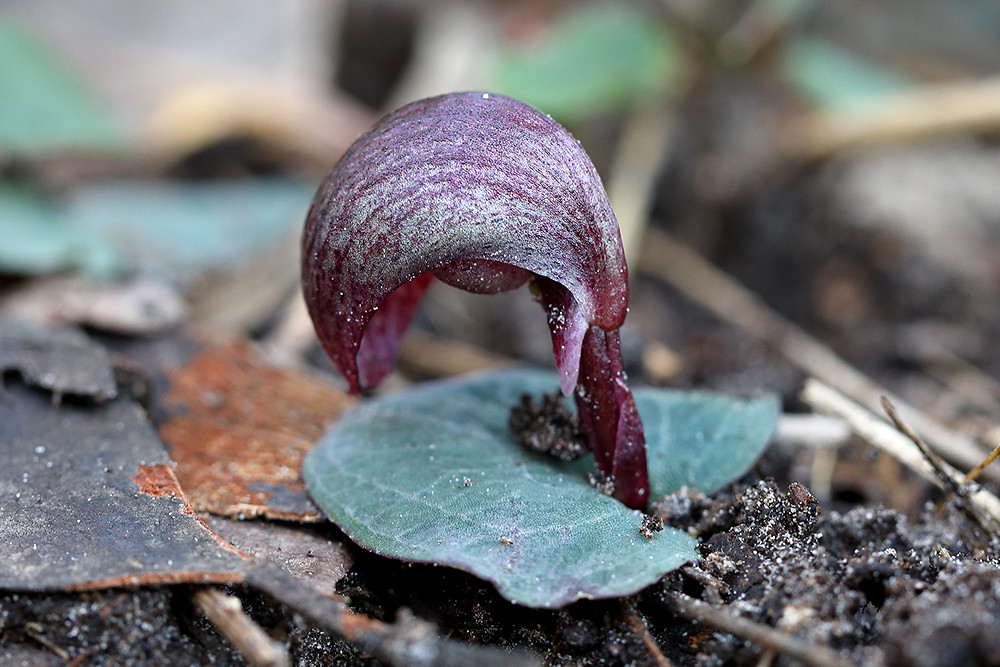In this detailed close-up photo, we observe a green leaf situated on a ground comprised of brown and black soil, with some orange debris visible on the left side. Emanating from the green leaf is a striking purple, almost burgundy-colored petal or part of the plant, which bends backwards to the left and exhibits a distinct moon-like shape. The foreground features a blend of black dirt with white specks and mulch-like chips interspersed with hints of orange. Surrounding the main subject, the backdrop is blurred, indicating a wooded or garden area filled with sticks, greenery, and additional dirt, which amplifies the focus on the intricately sprouting green leaf and its accompanying vibrant purple petal.